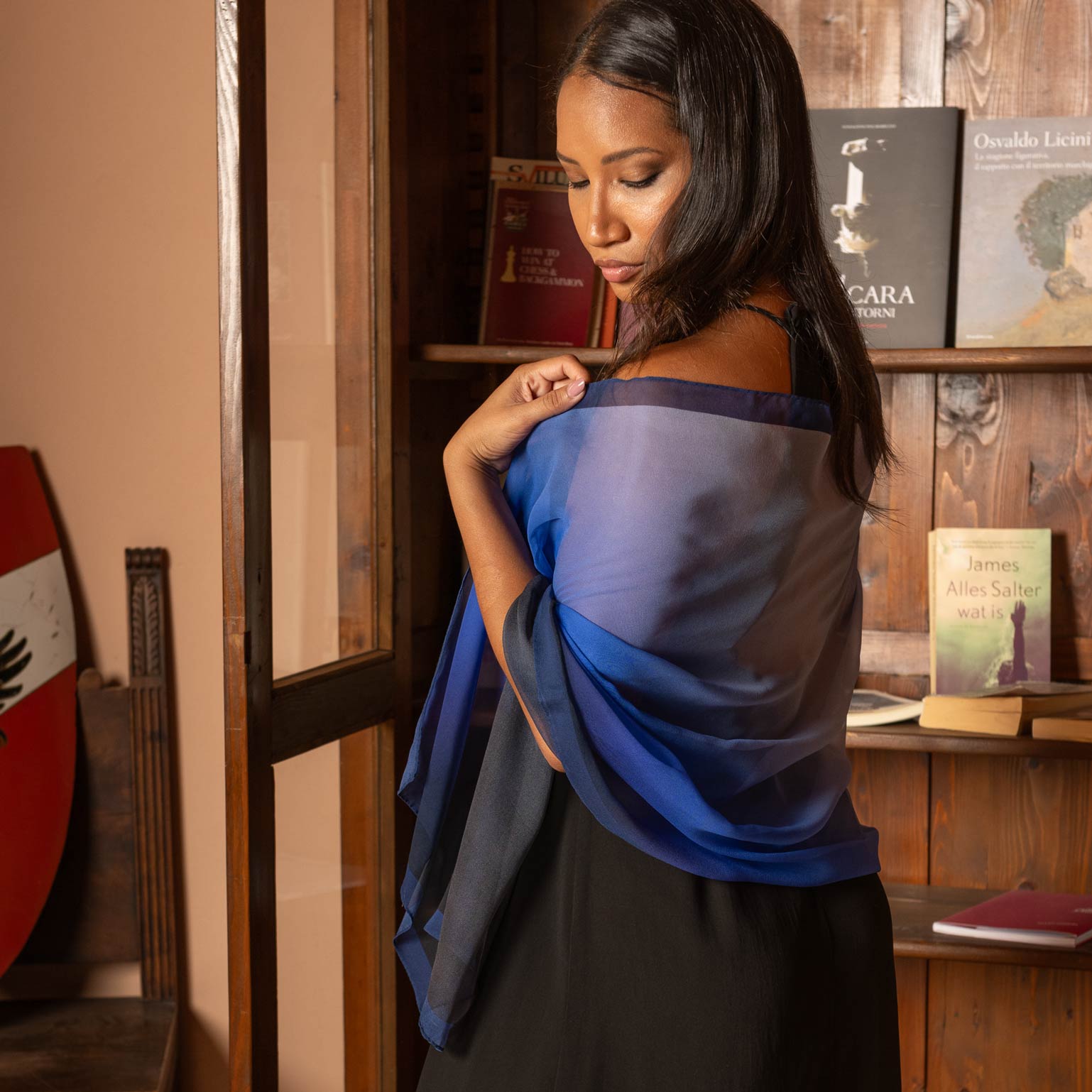The image features a striking young dark-skinned woman in her twenties, adorned in a black dress complemented by a slightly see-through dark blue shawl. Her long black hair cascades down as she stands with her head turned to the left, eyes closed, and appears to be looking down, possibly at the shawl draped elegantly over her arm and waist. The scene is set before a wooden bookcase with a few books on the shelves, not densely packed. One of the glass doors of the bookcase is open, showcasing books propped up for display, with titles like "Osvaldo Licini," "James Alice Salter," and "Guates" visible. To the left of her is a wooden section of the shelf, transitioning into an orange-tan wall. In the corner, an item resembling a big red crest with a white stripe and some intricate design sits, possibly on a chair, adding an element of mystery to the setting.